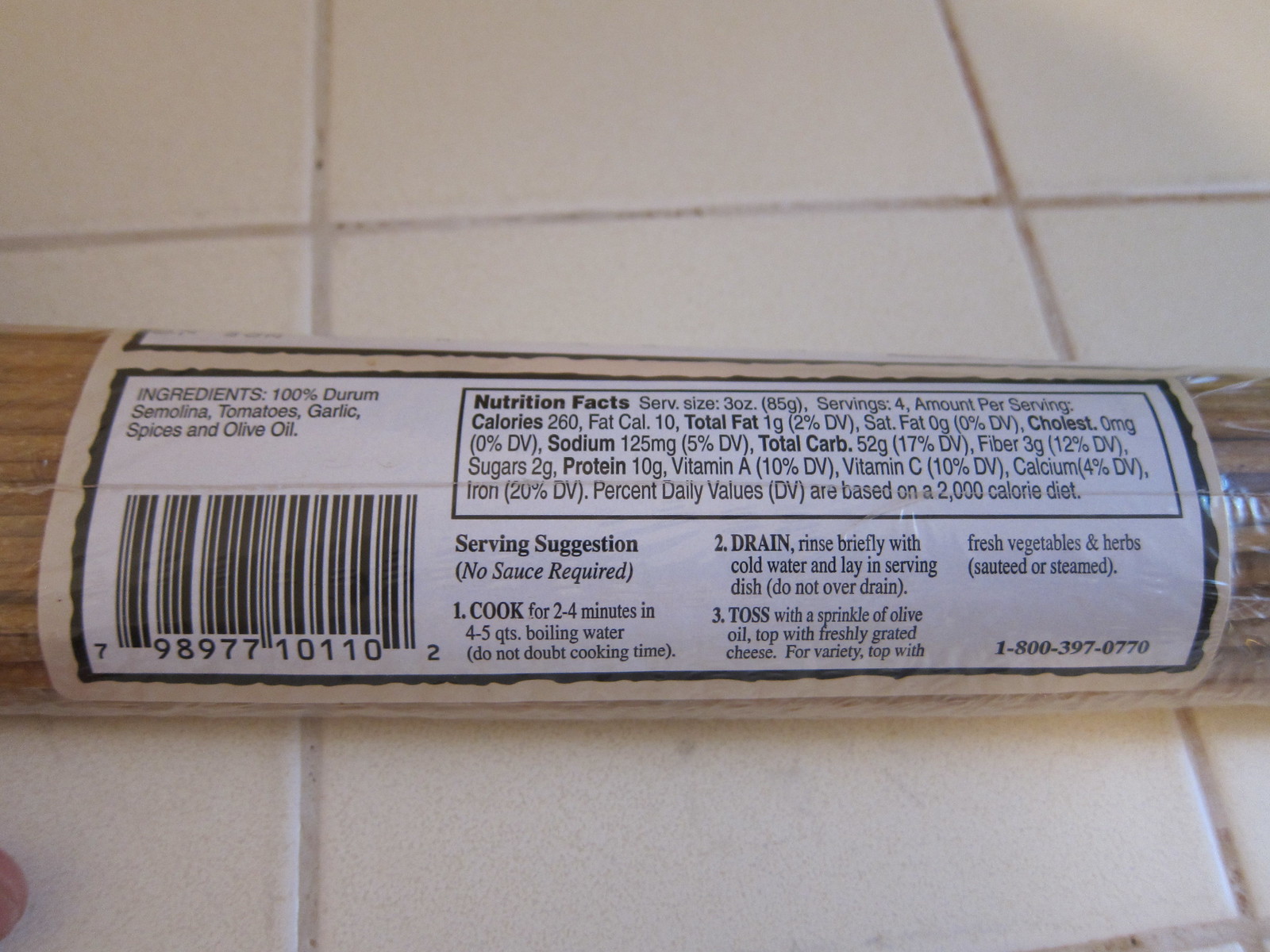This color photograph captures a clear cellophane-wrapped package of spaghetti laying horizontally on a dingy white tiled countertop with noticeable dirt in the grout lines. The spaghetti, made of thin strands of 100% durum semolina, is enwrapped with a package that prominently features a rectangular label. This label has a dark brown background with black printing, bordered by a lighter brown edge. On the top left of the label, there is an ingredients list: durum semolina, tomatoes, garlic, spices, and olive oil. Below the ingredients list sits a QR code. The right section of the label is dominated by nutritional facts in a bordered rectangle, taking up most of the right side. Below the nutritional information, there is a "serving suggestion" section stating: "Cook for two to four minutes in boiling water, drain, toss with a sprinkle of olive oil." In the bottom right corner of the label, there's a customer service contact number. The detailed printing on the label provides thorough product information, making it clear for consumers.